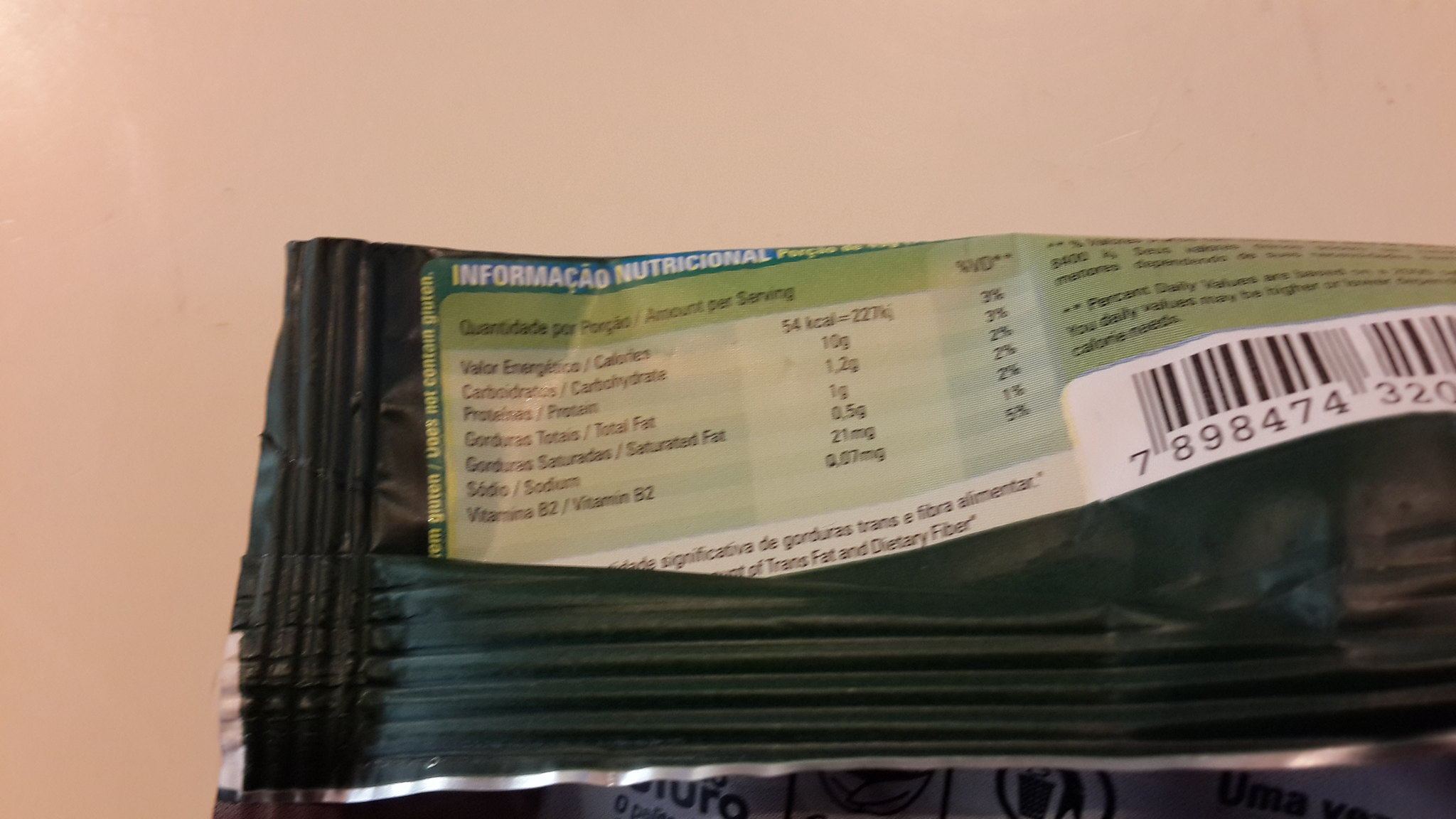This color photograph depicts a close-up of several black plastic or paper labels organized in a neat stack against a muted peach or orange-tan background. The labels are printed in another language, potentially Spanish or Portuguese, with "Información Nutricional" prominently displayed at the top, outlining the nutritional content of a food product. The label features various shades of green and includes detailed information such as calorie count (94 calories) and other dietary specifics. A distinct black-and-white barcode with the numbers 7898474320 is located towards the left side of the label, while a narrow silver band runs along the bottom. The scene is faintly illuminated from the upper left corner, adding slight shadows and enhancing the details of the textured surface under the labels. The overall composition suggests a professional packaging setup, designed for retail display.